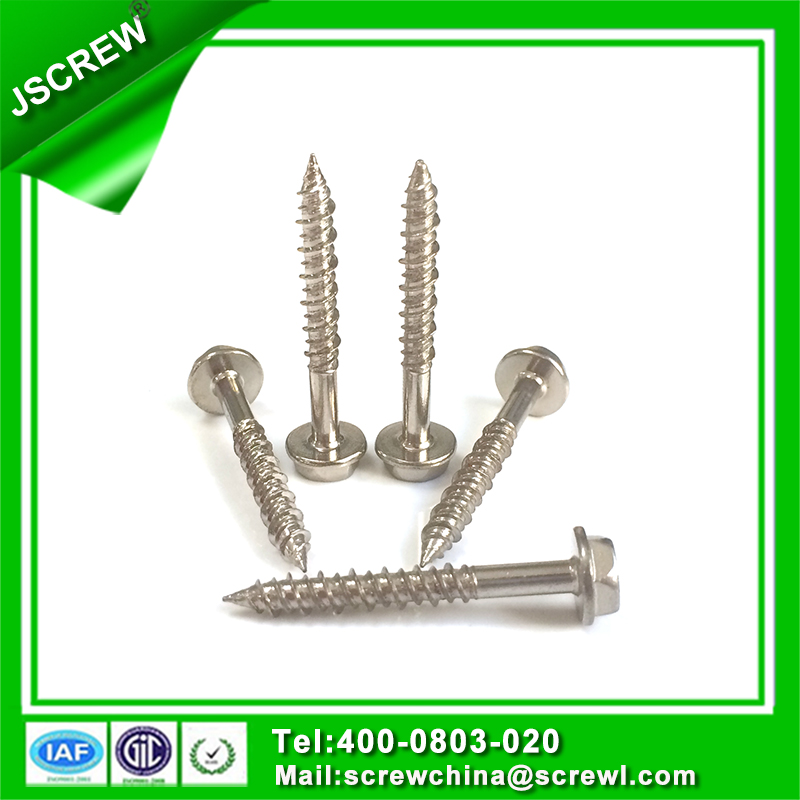The image is a promotional ad with a green border and white inner border, featuring a central white square with five silver screws arranged inside it. Two screws stand upright near the center, flanked by two screws lying down diagonally, with a fifth screw positioned horizontally in front. In the upper left corner, "JS Screw" is written in white font against the green border. At the bottom left, three small logos are displayed, followed by the text "Telephone 400-0803-020" in white font. Below this, the contact email "screwchina@screwdell.com" is provided. The top right-hand corner has a folded-over effect. The overall image serves as a detailed and organized promotional layout for screws.